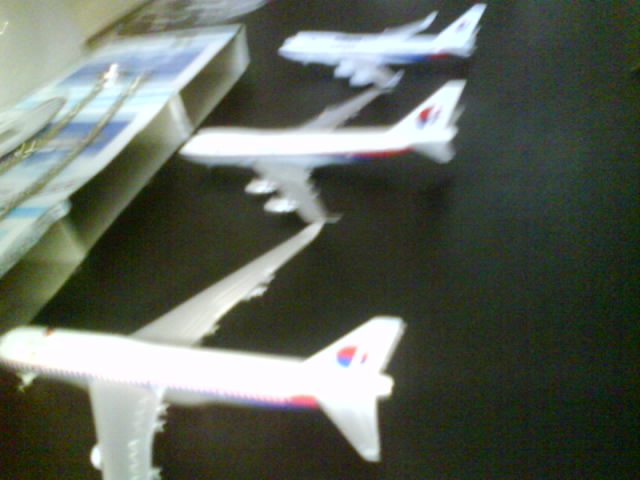A top-down photograph captures three white model commercial airliners with gray wings, arranged in a row on a solid black floor. The models, distinguished by blue and red semicircles on their tails and similar markings on their bodies, have their wings positioned closely as if nearly touching. The background features an unclear structure, likely boxes or a cloth-covered table, positioned to the left with three openings. A long metal object runs vertically alongside the floor in the image. The overall scene is extremely blurred, obscuring finer details and making it difficult to distinguish specific elements clearly.